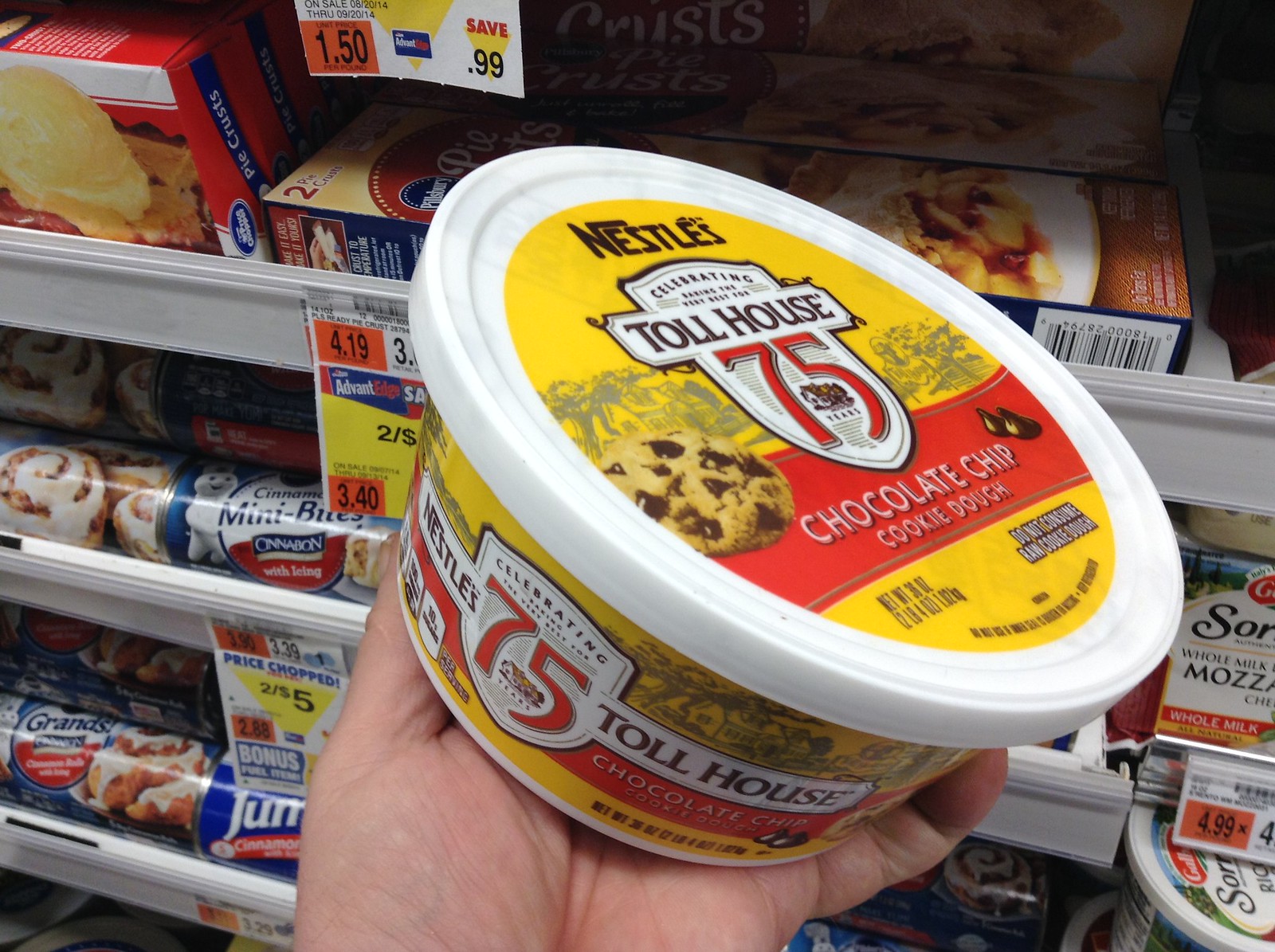This photograph captures a close-up view of a person's hand holding a round container of Nestle Tollhouse chocolate chip cookie dough in what appears to be a grocery store's refrigerated section. The container stands out with its distinct design: a white base adorned with a yellow label featuring a prominent red banner that reads "celebrating 75 years." The Nestle Tollhouse logo is clearly visible, and the lid mimics this yellow and red design. Behind the hand, the store shelves are stocked with various refrigerated items such as cinnamon rolls, pie dough, grahams, mini bites, and cheeses, highlighted by price tags that hang along the shelves. This image emphasizes the commemorative aspect of the product packaging, celebrating 75 years of Tollhouse cookies.